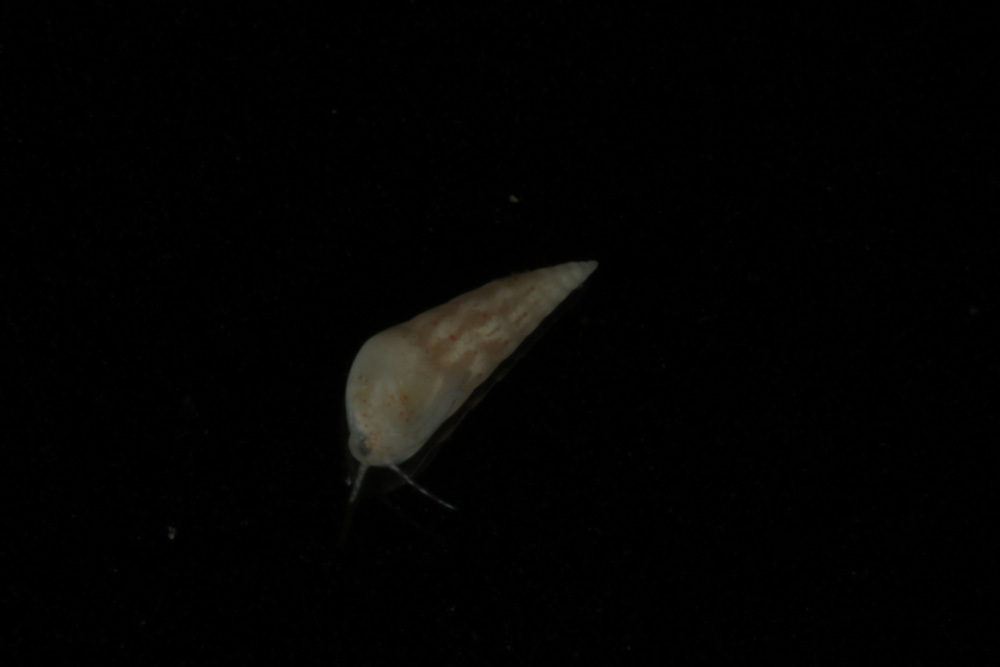Amidst an almost entirely pitch-black background speckled with a few subtle dots, a mysterious sea creature occupies the central left portion of the image. The creature, which is primarily cone-shaped, features a narrow, ribbed tail that extends from the northwest of the frame to the wider front end positioned towards the southwest. This wider section appears to host an eye or orifice, potentially used for feeding, along with two antenna-like appendages. The body of the sea creature is brown and exhibits a striped pattern towards its tail, evoking a resemblance to a caterpillar. Despite its somewhat gelatinous appearance, there is an implication of a shell-like texture covering its elongated form. The absence of context, enhanced by the pitch-black backdrop, leaves the nature of the creature's environment—whether floating or resting on a surface—ambiguous. The image, blurred slightly, carries the aesthetic of nature photography, capturing the enigmatic essence of this unusual marine life.